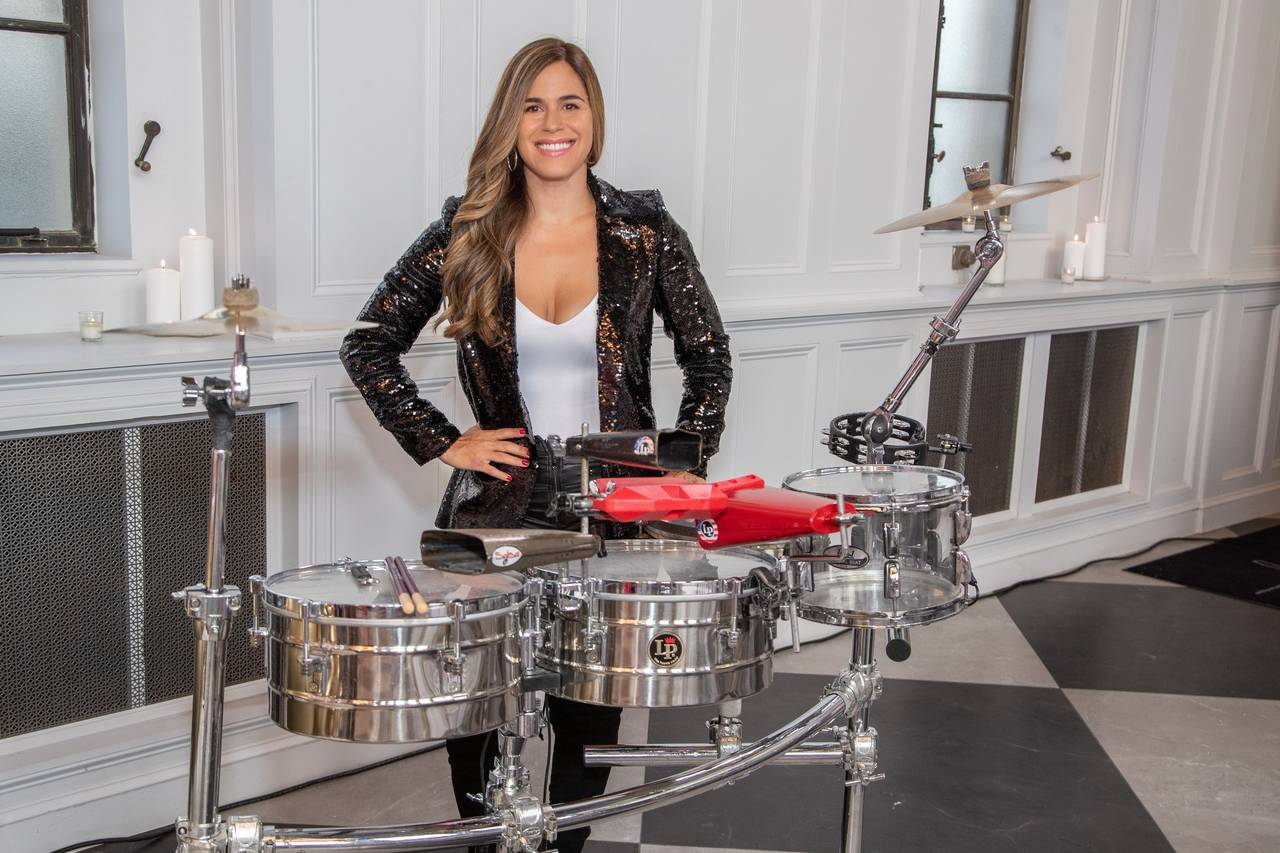In a largely white room with some grates and opening windows at the top, stands a young woman in her 20s or 30s, fair-skinned with flowing golden brown hair cascading over her right shoulder. She is beaming directly at the camera, a big smile brightening her face. Dressed in a sparkly dark jacket with gold and silvery embellishments, a low-cut white tank top, and black leather pants, she exudes confidence with her hands placed firmly on her hips. Behind her is a silver drum set emblazoned with an "LR" symbol, featuring multiple cymbals, three drums, red and black cowbells, and visible drumsticks. The floor beneath her feet resembles a giant chessboard with alternating black and white polyhedron tiles. The white walls behind her hold white candles, adding a soft glow to the serene ambiance.